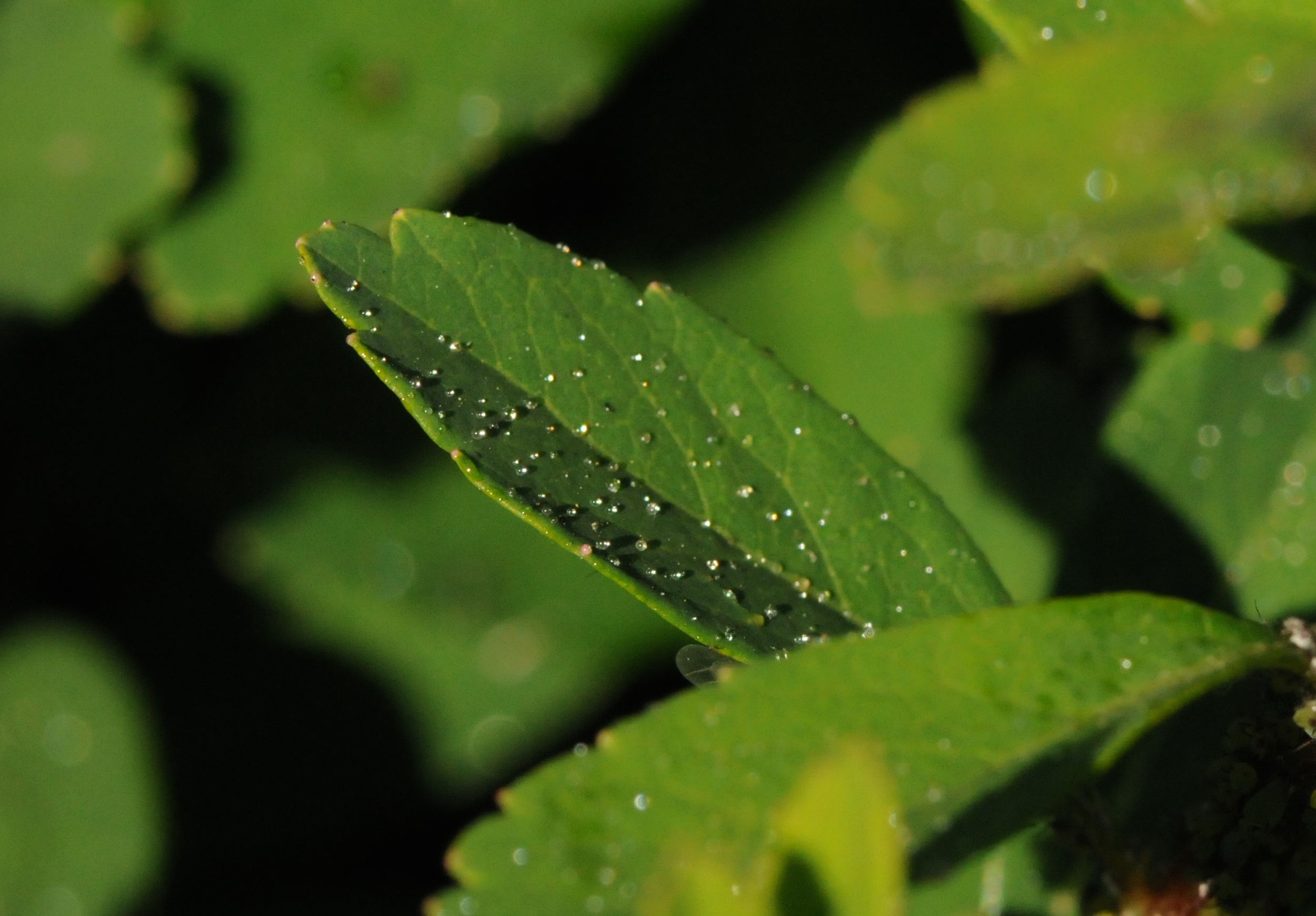The image showcases an extreme close-up of a single, prominent green leaf with jagged edges and detailed veins, covered in numerous dew droplets. The leaf, which transitions from a lime green on the right to a darker green on the left, appears exceptionally sharp and clear against a blurred background of other leaves. These background leaves, also sprinkled with dew, are visible but not in sharp focus. The scene suggests a post-rain environment, with the black sky adding a contrasting backdrop to highlight the detailed textures and vibrant greens of the leaves.